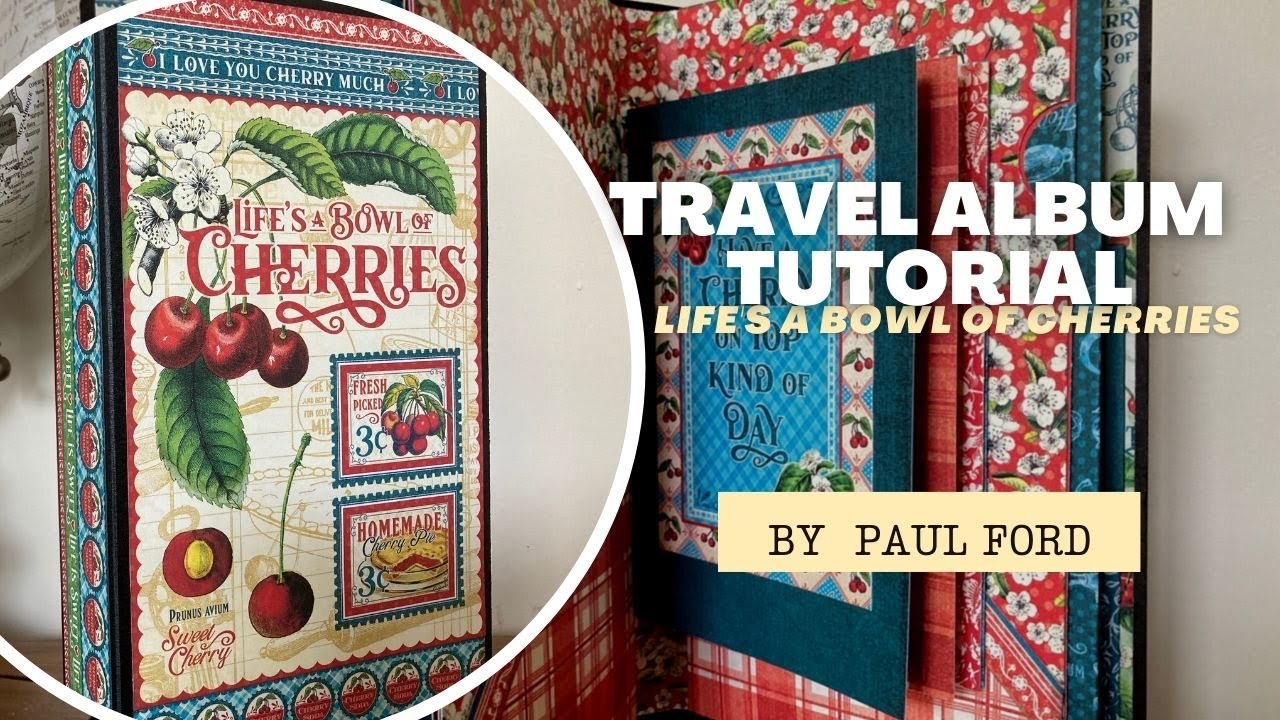The promotional image showcases a tapestry-like background with rich red and flower motifs, evoking a vintage charm. Central to the image is the title, "Travel Album Tutorial, Life's a Bowl of Cherries by Paul Ford," featured prominently on the right side. This area seems to depict a framed picture against a red wallpaper decorated with white flowers. A circular inset on the left side highlights the cover of a book titled "Life's a Bowl of Cherries," with text reminiscent of old-timey, Coca-Cola-like lettering in looping red script. The cover features vivid illustrations, including cherries with green leaves and additional decorative stamps. One stamp shows cherries with the label "Fresh Pick, 3 cents," while another displays a cherry pie with the caption "Homemade Cherry Pie, 3 cents." A cherry pit illustration in the bottom left corner of the inset is marked "Picked with Sweet Cherry," adjacent to a single cherry. The composition of the image blends elements to create a nostalgic and cohesive visual narrative.